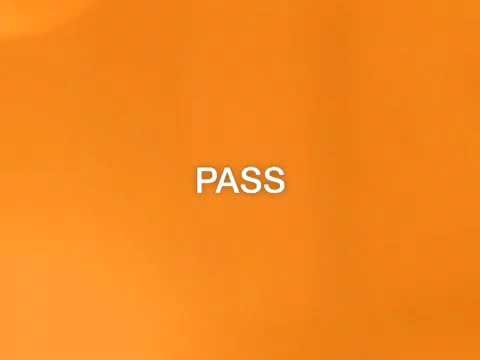The image is a square with a vivid, bright orange background. In the middle of this solid orange square, the word "PASS" is prominently displayed in all capital letters. Each letter of "PASS" is white, simplistic, and easy to read. Despite the orange background being mostly solid, subtle streaks of lighter and darker shades of orange can be observed. There are no other images, words, or references present, making the design very minimalistic and straightforward.